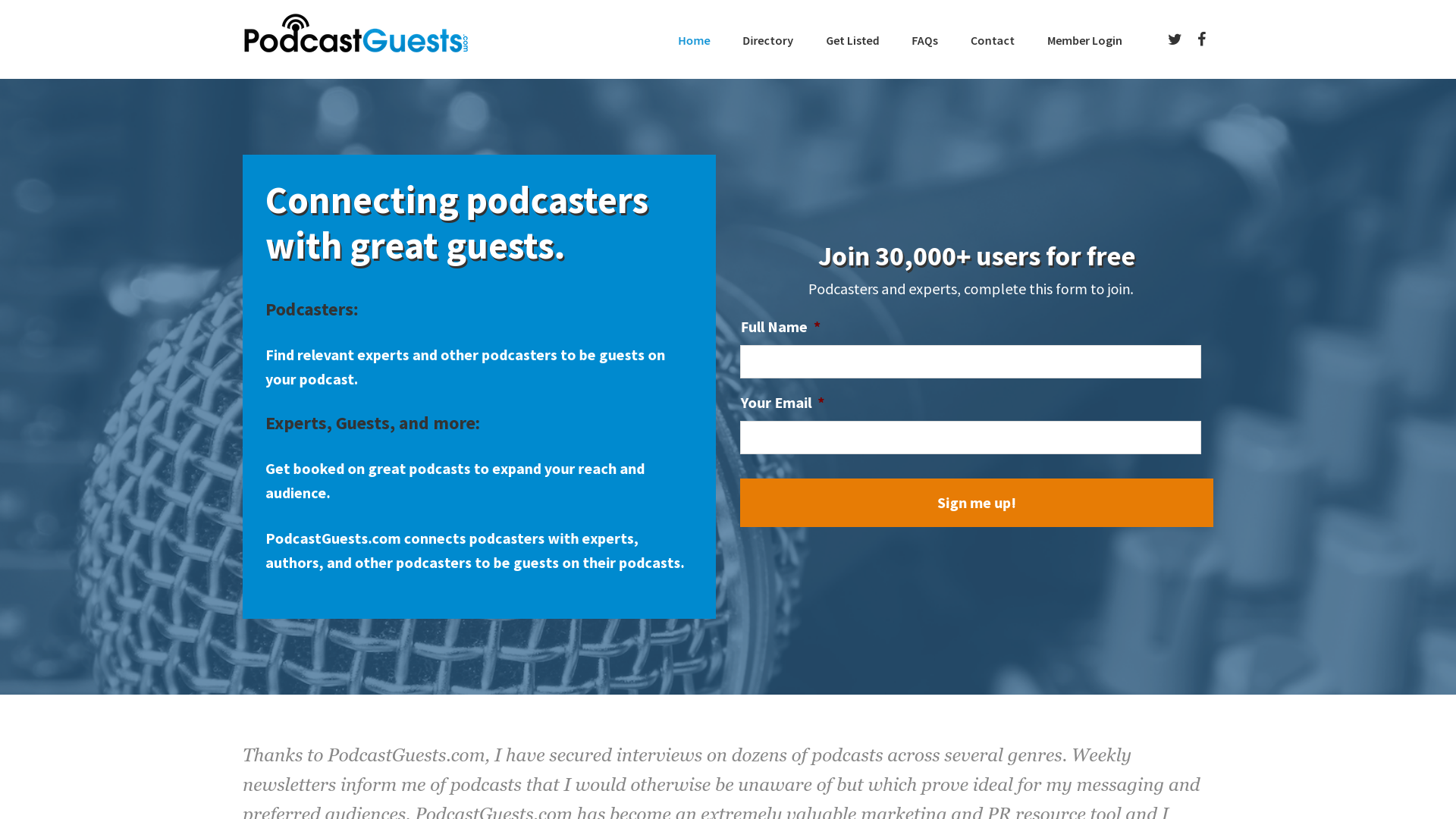The image displays a screen capture of a website viewed on a desktop computer. The screen features a gray background, which is actually a blurred image of a microphone’s mesh head, depicting the intricate crisscross pattern and circular shape typically seen on professional microphone heads.

Prominently in the foreground, there is a vibrant blue square with bold white text that reads, "Connecting Podcasters with Great Guests." Below this main headline, additional text in black and white provides further details.

To the right of the blue square, white text announces, "Join 30,000 Users for Free. Podcasters and Experts Complete the Form to Join." Beneath this text, a registration form is visible, consisting of two white text boxes designed for user input. Directly below these input fields, an eye-catching orange button with the inscription “Sign Me Up” in white text invites users to register.

The overall design effectively draws attention to the call-to-action and registration process, combining professional aesthetics with clear instructions.